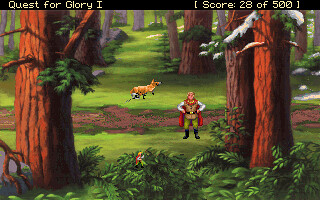This image is a pixelated screenshot from the early 1990s PC game "Quest for Glory 1," as indicated by the game title in the top left corner and a score of 28 out of 500 displayed beside it. The scene depicts a character in the center, dressed in a Robin Hood-like outfit consisting of green pants, black boots, a white long-sleeve shirt, a brown vest, and a red cape. The character is blonde, although the pixelation obscures facial details. They stand in a forest setting, surrounded by tall, large trees varying in color from dark brown to reddish and light brown. Pine trees with patches of snow on their leaves frame the path that cuts through the scene from right to left. At the character's feet, along the dirt path, are sprigs of greenery and bushes. A notably orange and white fox with black feet appears to the upper left of the character, while a small red parrot or frog is nestled in the bushes at the bottom of the image, adding vibrant touches to the otherwise earthy and green-toned landscape.